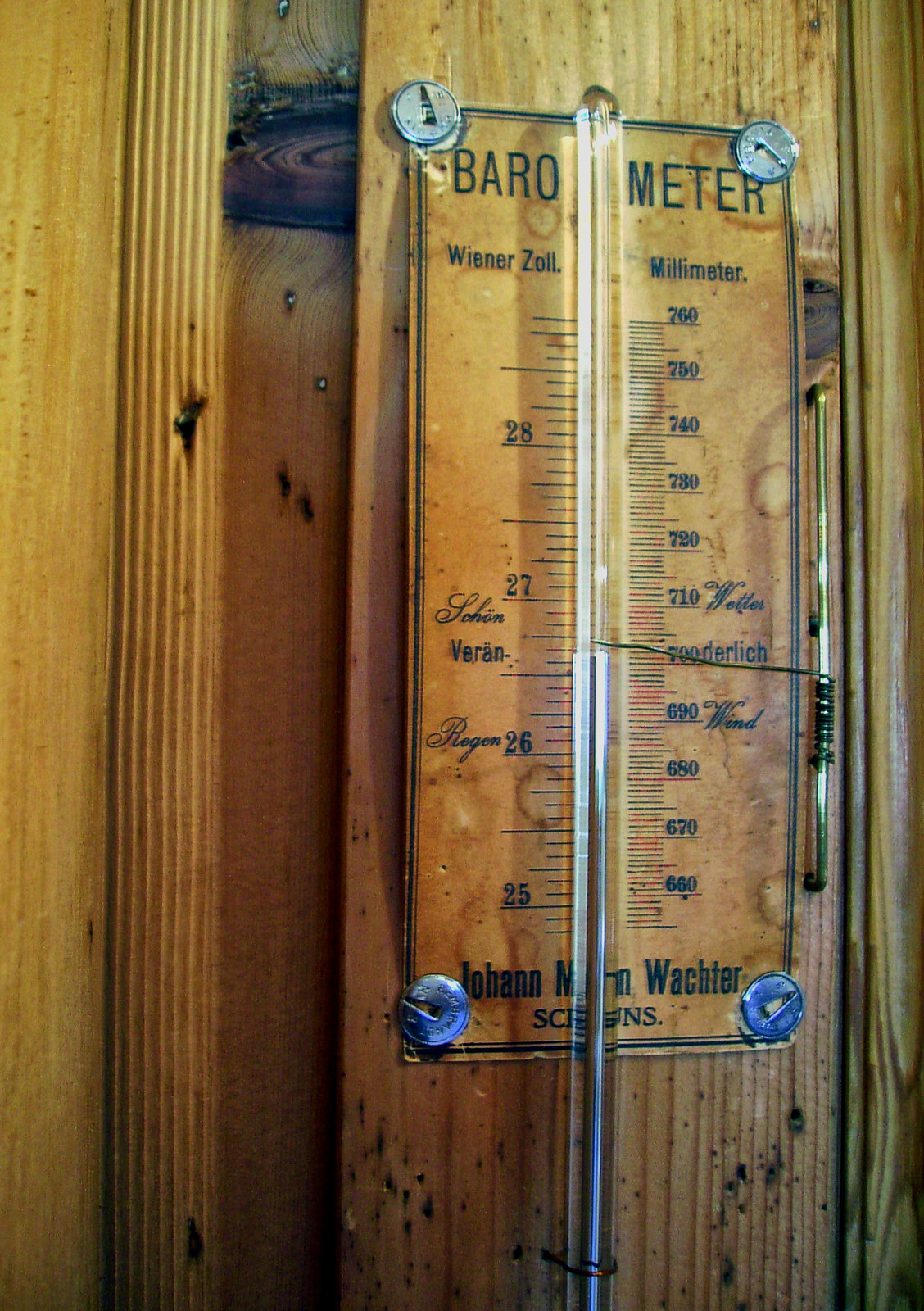The photograph features a wooden barometer, securely attached to a wooden wall with silver circular fasteners at all four corners. The instrument, crafted with a polished brown finish, merges traditional and elegant designs. Black inscriptions and numerals adorn its surface, providing readings in both German and millimeters. A transparent, thermometer-like tube runs vertically through its center, highlighting its dual functionality. On the right side, the scale starts at 760 millimeters at the top and descends incrementally with markings at 750, 740, 730, 720, 710, 700, 690, 680, 670, and 660 millimeters. On the left side, measurements decrease from 28 down to 25 units. The bottom of the barometer is inscribed with the barely legible name "Johann Bächter" or a similar German name, hinting at the manufacturer's identity.